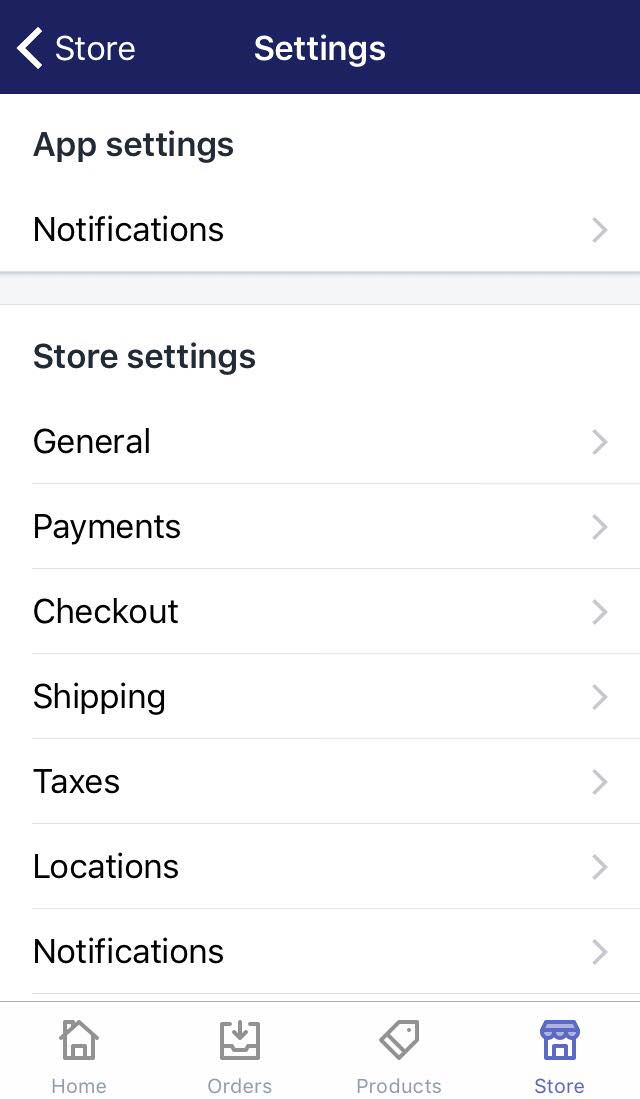The image depicts a laptop screen displaying a dashboard interface focused on an e-commerce platform. At the top, there's a navy blue banner with white text showing "Store" on the left and a highlighted "Settings" section. Below the banner, the screen is divided into a white-background menu with various settings categories. 

The primary sections visible include:
- "App Settings" in bold black text.
- "Notifications" marked with an arrow indicating it can be expanded for further options.

Under the "Store Settings" with a darker font, there are several expandable categories, each accompanied by an arrow:
1. General
2. Payments
3. Checkout
4. Shipping
5. Taxes
6. Locations
7. Notifications

At the bottom of the screen, there are navigational icons paired with text labels:
- A house icon labeled "Home"
- A stack of papers labeled "Orders"
- A tag icon labeled "Products"
- A storefront icon labeled "Store," which is currently selected, indicating the user is viewing the store settings.

This comprehensive interface allows for detailed customization and management of various store aspects, highlighted by the active section on the screen.